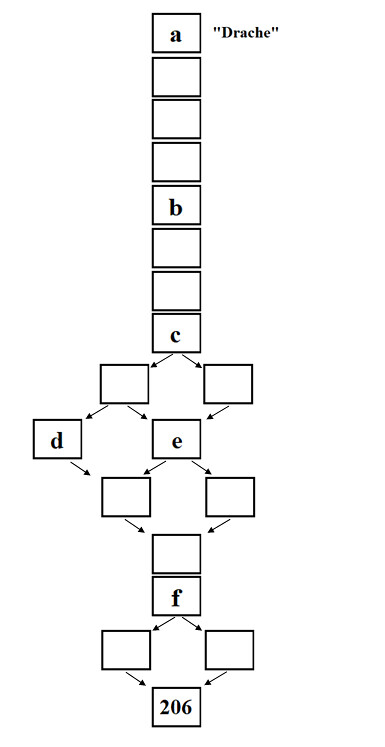The image displays a structured flowchart composed of a series of black, empty boxes on a white background, arranged to depict a hierarchical relationship. Here is a detailed description:

1. **Top Row**: It starts with one box at the top labeled 'A'. To the right of this box, outside of the main structure, the word "Trash" is written in quotation marks.
2. **Second to Fourth Rows**: Directly below 'A', there are three consecutively empty boxes forming a vertical column.
3. **Fifth Row**: The box in this row is designated 'B', followed by two vertically aligned empty boxes beneath it.
4. **Eighth Row**: The next box down is labeled 'C', branching into two separate empty boxes below it. Arrowed lines extend from 'C' to these two side-by-side boxes.
5. **Tenth Row**: In this row, two horizontally aligned boxes are marked 'D' on the left and 'E' on the right. Arrows connect these boxes to the previous level's respective boxes.
6. **Twelfth Row**: Beneath the 'D' and 'E' row, two empty boxes are connected by arrows, converging into one single empty box below them.
7. **Fourteenth Row**: This singular bottom-center box is labeled 'F', which further splits into two empty side-by-side boxes below it with arrows directing the path.
8. **Sixteenth Row**: The final row features a single central box labeled '206', connected by arrows from the two previous boxes.

The overall layout suggests a procedural or decision-making flowchart, though its exact purpose remains unclear.